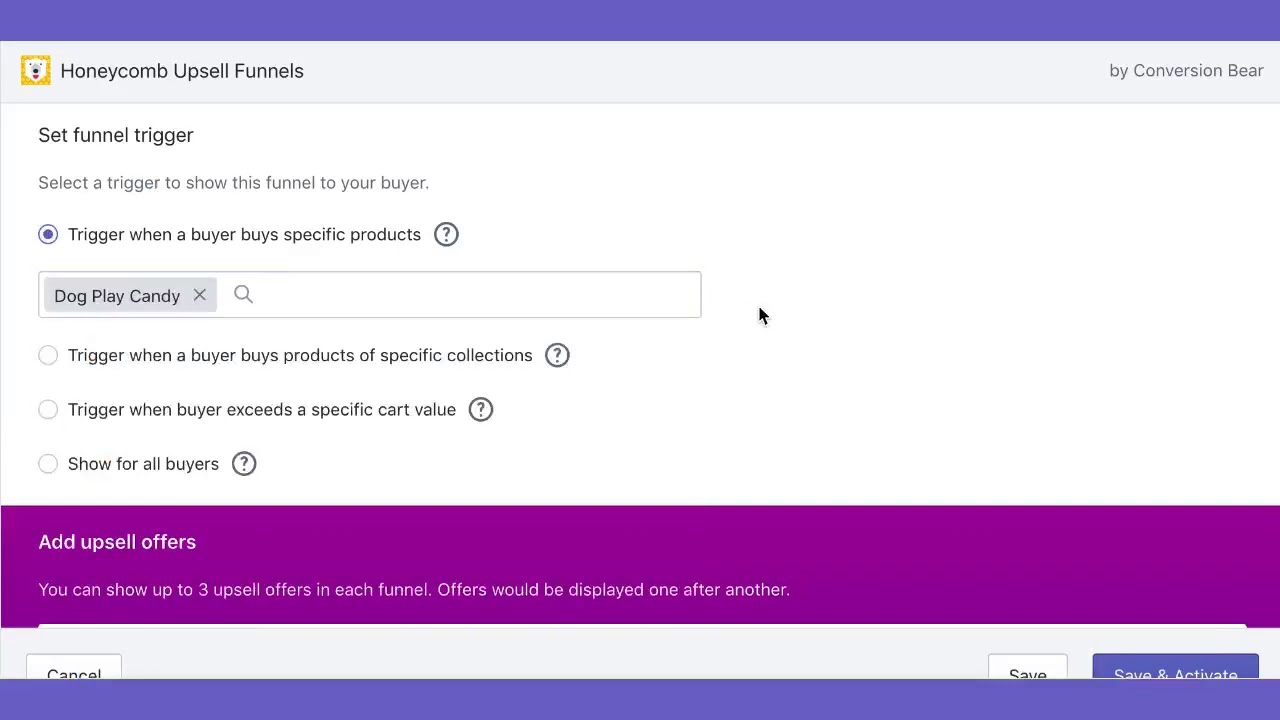This is a website interface detailing the setup process for Honeycomb Upsell Funnels, with the prominent Conversion Bear logo featuring a bear icon. The page allows users to configure funnel triggers to display upsell offers to buyers.

### Page Layout:

- **Top Section:**
  - **Logo:** Bear logo representing Conversion Bear.
  - **Title:** "Honeycomb Upsell Funnels".

- **Middle Section:**
  - **Instructions:** "Set Funnel Trigger" followed by a prompt to select a trigger to display the funnel to buyers.

- **Trigger Options:**
  - A check-marked bubble option reading, "Trigger when a buyer buys specific products", accompanied by a question mark icon for additional information.
  - Additional trigger options in vertical bubbles:
    - "Trigger when a buyer buys products from specific collections" (with a question mark icon).
    - "Trigger when a buyer exceeds a specific cart value" (with a question mark icon).
    - "Show for all buyers" (with a question mark icon).

- **Tags and Search:**
  - A tag marked "dog play candy" with an option to close.
  - A search bar for finding specifics within the process.

- **Banner:** A purple banner stating, "Add upsell offers. You can show up to three upsell offers in each funnel. Offers will be displayed one after another."

### Bottom Section:

- **Buttons:**
  - **Left:** "Cancel" button.
  - **Right:** "Save" button and "Save and Activate" button.

- **Footer:** Another purple banner similar to the one above.

This detailed setup walkthrough is designed to help users configure their upsell triggers effectively within the Honeycomb Upsell Funnels tool by Conversion Bear.